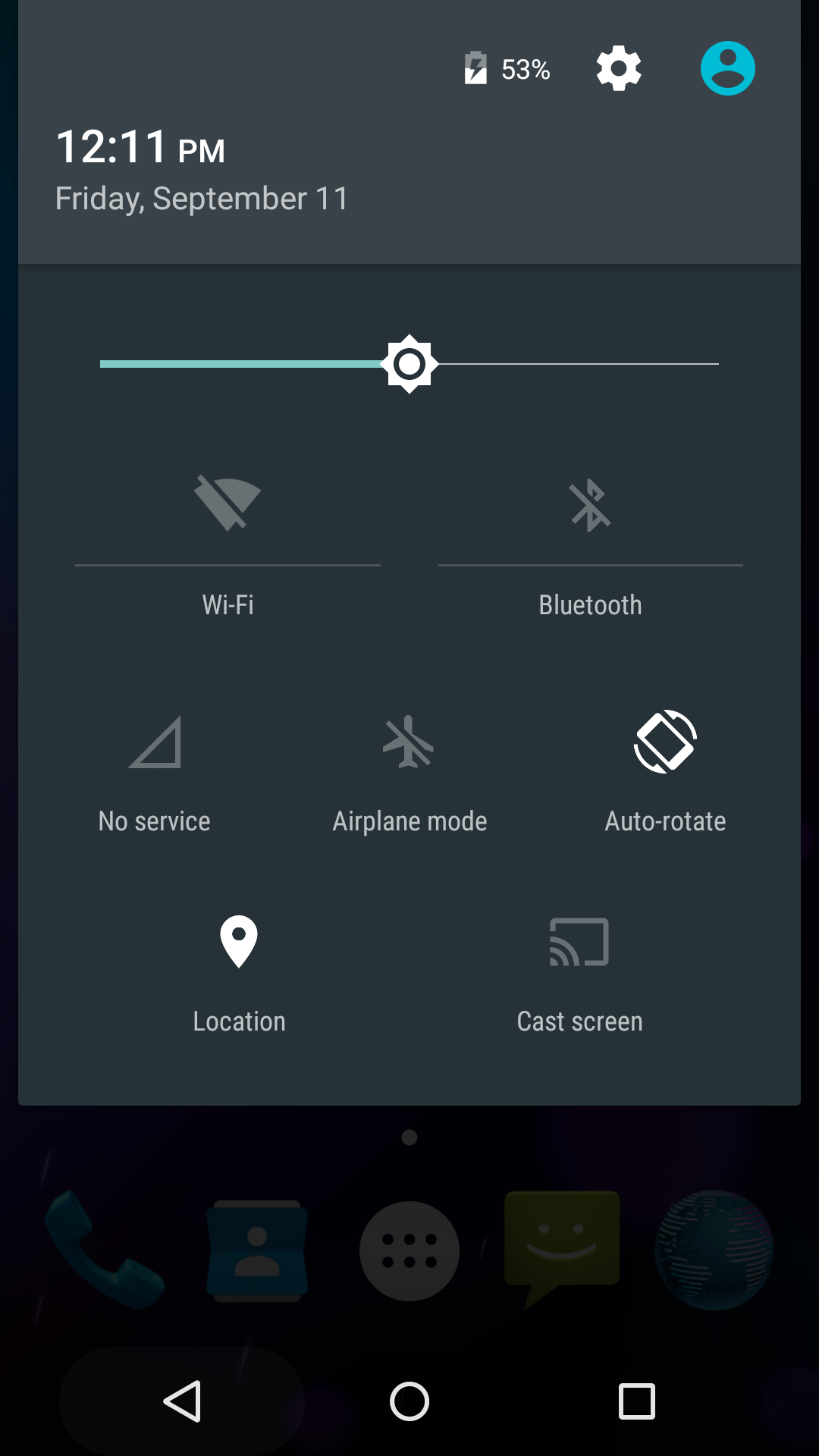The image depicts a screenshot of an Android phone displaying its settings menu. The phone features a black or navy blue theme. At the bottom of the screen, the familiar navigation icons of triangle, circle, and square are visible, signifying it is an Android device.

At the top of the screen, the date and time are shown as Friday, September 11th, 12:11 PM. To the right, the battery indicator displays a 53% charge with a lightning bolt symbol, indicating that the phone is charging. Next to the battery icon, there is a settings wheel and a user icon.

The pull-down settings menu is halfway down, revealing various quick access buttons and options. The brightness slider is visible, suggesting that the user might be adjusting the screen brightness. The Wi-Fi and Bluetooth icons are both displayed as turned off. The service status indicates "No service." Airplane mode is not activated, while auto-rotate and location services are enabled. The cast screen option appears to be turned off.

In the blurred background, the faint silhouette of the home screen menu can be seen, hinting at the user's ongoing adjustment of settings on their Android device.